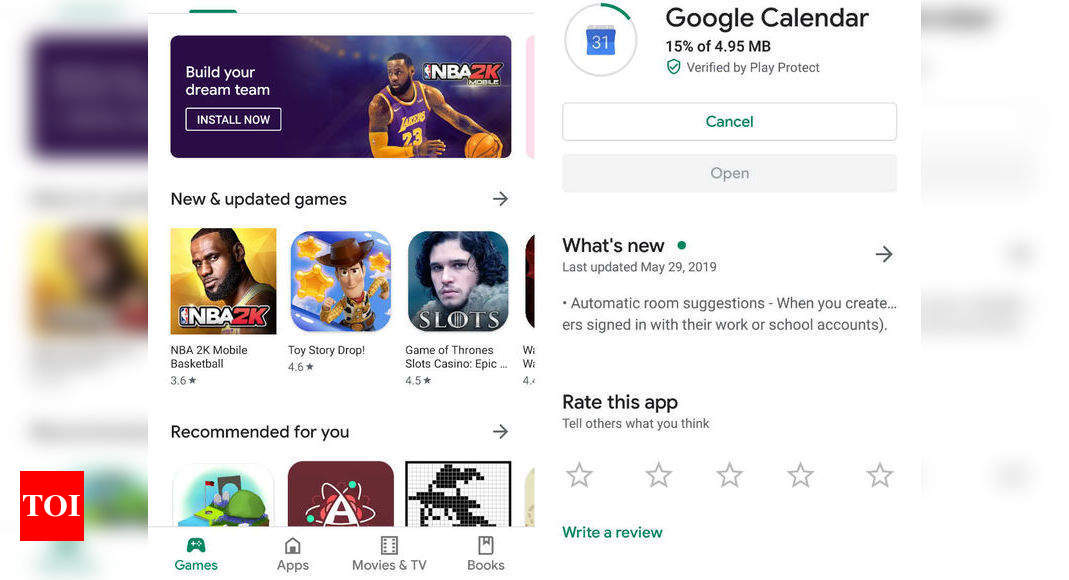This is a detailed caption for the given image:

---

The image is a screenshot capturing a dialog box interface from the Google Play Store against a blurred background. On the left column, there are several blurred-out images, likely previews of the apps or games featured in the dialogue, adding a layer of visual content but remaining indistinct. In the bottom left corner, a red and white rectangle prominently displays the text "TOI." 

At the top of the dialog box, a promotional message encourages users to "build your dream team" and urges, "install now NBA 2K." Beneath this banner, a section labeled "new and updated games" features a list of titles including NBA 2K, Toy Story Drop, Game of Thrones Slots Casino, among others.

Further down, the interface transitions into a "recommended for you" section showcasing various icons representing games, applications, movies and TV shows, and books. However, a portion of this section is obscured by a dialog displaying the download progress of the Google Calendar application, which indicates it is 15% complete. The progress circle visually represents the ongoing download. This image captures a moment within the active use of the Google Play Store, highlighting both a promotional feature and a simultaneous app download.

---

This detailed description provides a thorough breakdown of the elements present in the screenshot and their arrangement.